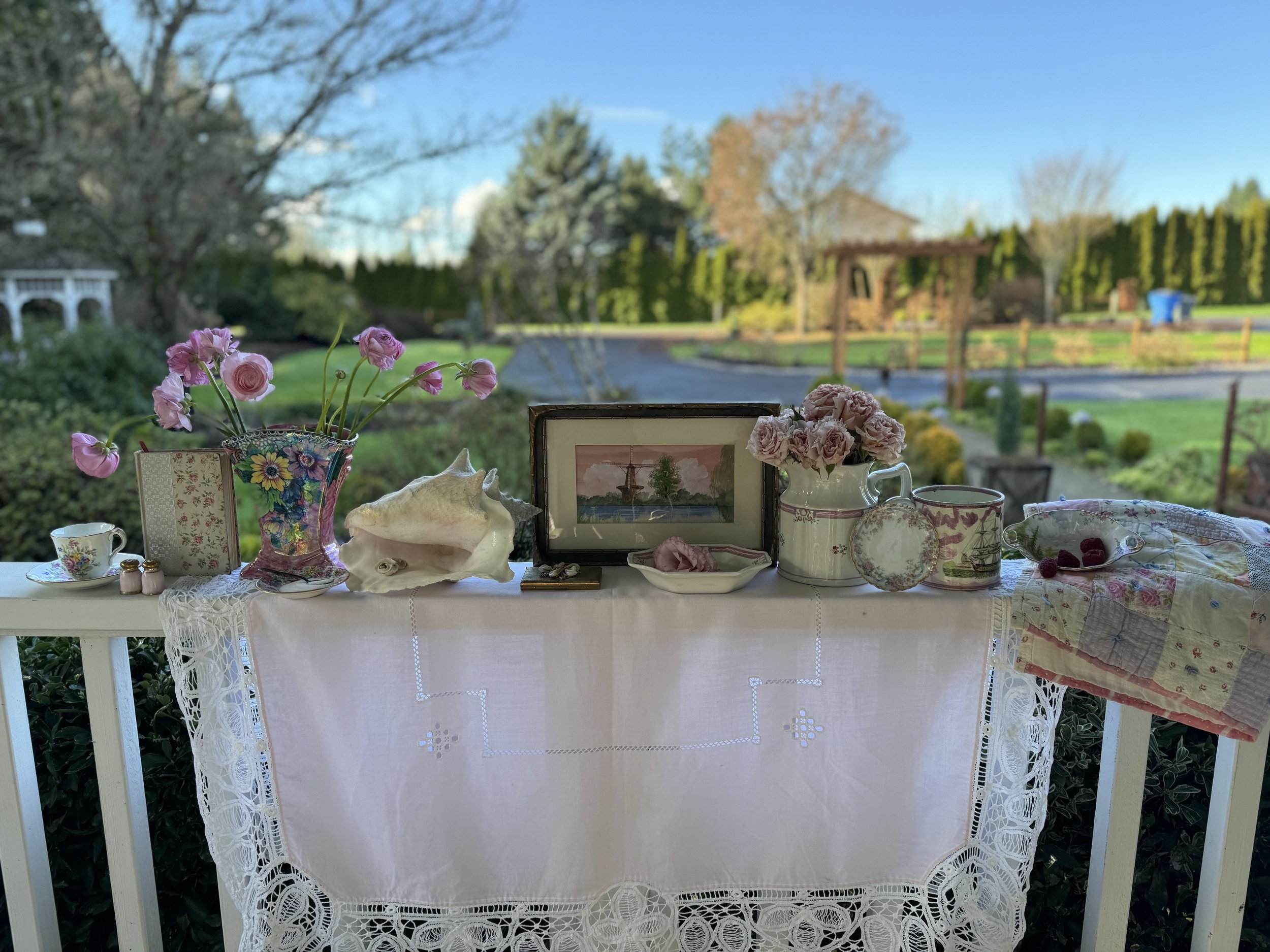This image captures an elegant setup on the side of someone's porch, featuring a white railing adorned with various decorative items. Draped over the railing is a white tablecloth with a lacy, doily-like border. The display includes a charming arrangement of feminine items: starting from the left, there's a teacup and saucer set, a small salt and pepper shaker, a decorative box, and a flower vase filled with pink and purple roses. A large white seashell rests next to a framed illustration depicting a serene pink sky over water, bordered by a white mat and frame. Further along, there's a pitcher filled with roses, assorted plates and mugs, a small ceramic container with a lid, and a bowl that appears to contain raspberries. In the background, the natural setting features a lush green landscape with large trees, a manicured lawn, a little gray road or driveway, and a picturesque white gazebo. The scene exudes a sense of tranquility and refined taste, framed by the pristine, white-painted wooden porch railing.